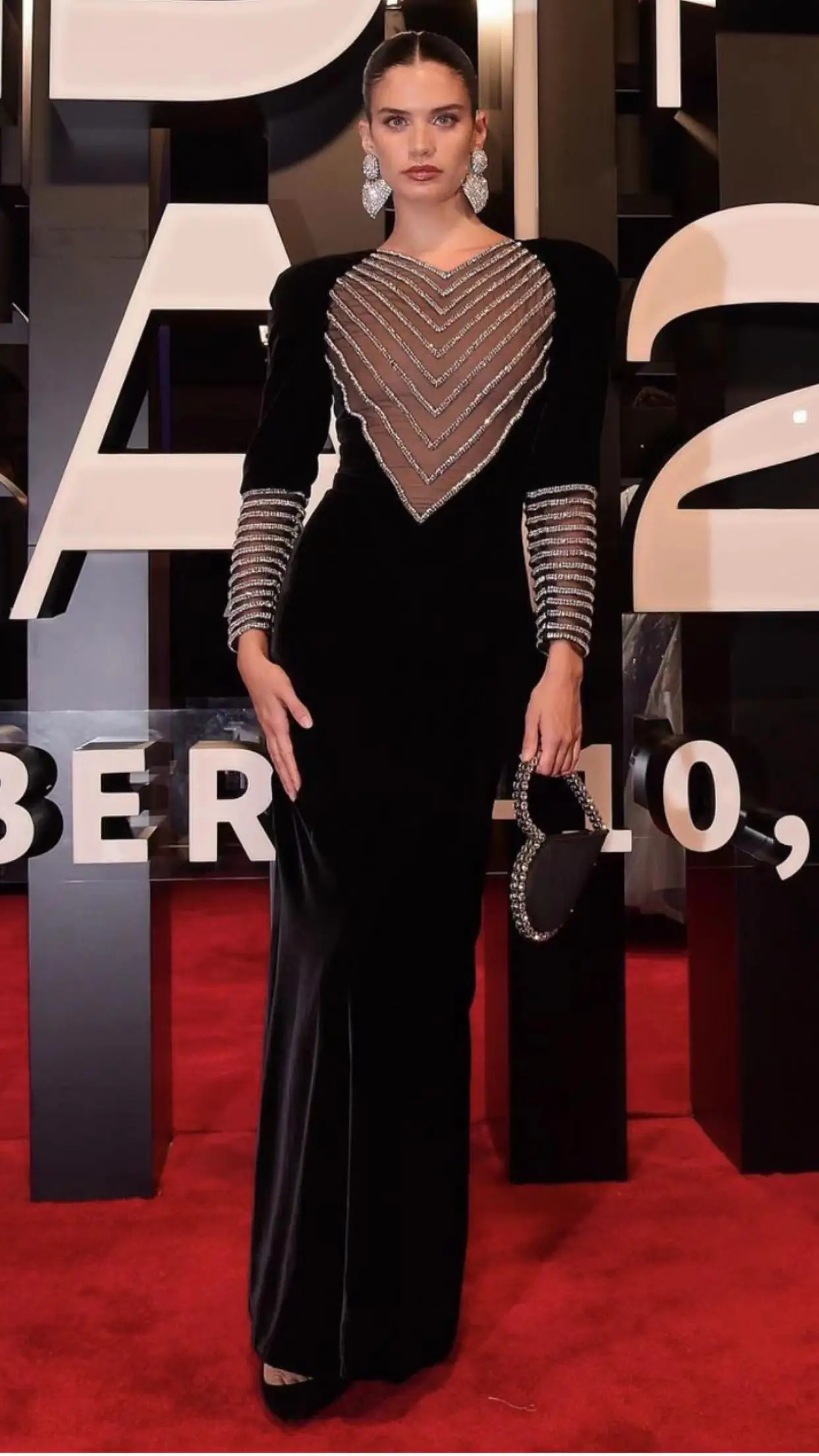In the image, we see a woman, possibly an actress or model, standing and posing on a plush red carpet. She is wearing a striking black gown with intricate details. The gown features a heart-shaped, see-through section on the chest adorned with glittery silver lines, allowing a peek at her skin. The sleeves of her gown are also sheer, covered from the wrist to the elbow with sparkling silver rings, adding a touch of elegance. She has her dark hair pulled back into a sleek ponytail with a middle part, accentuating her carved eyebrows and full red lips. Her look is completed with large, diamond-encrusted earrings that are heart-shaped at the bottom and round at the top, adding a bold statement. She carries a small heart-shaped purse and though her black shoes are mostly hidden by the long gown, they contribute to her polished appearance. The background features bold white text and numbers, though they are not clearly distinguishable, and the surrounding lights create reflections and cast shadows, enhancing the ambiance of the red carpet event.